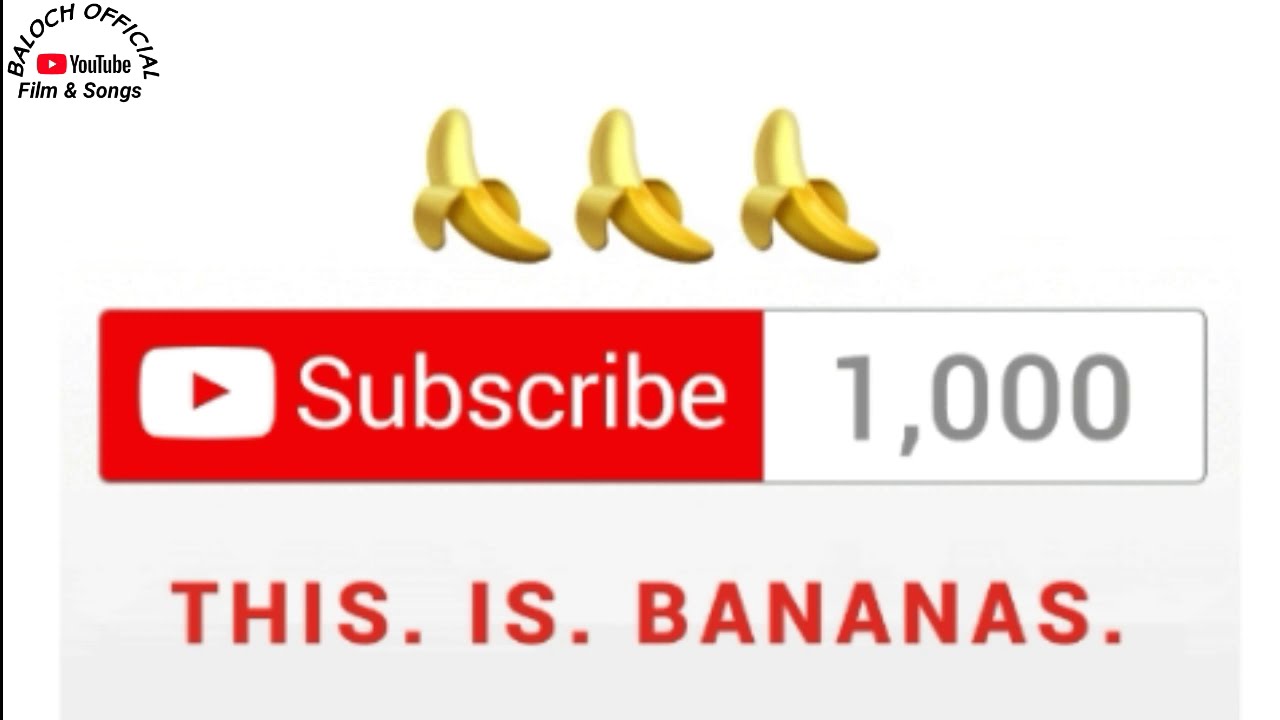The image features a prominent YouTube subscribe button in the center against a gradient gray background, darkening from top to bottom. Above the button, three symbolic, half-peeled bananas are aligned horizontally. Below the bananas, the subscribe button is depicted within a red rectangle, featuring the YouTube Play logo (a white triangle in a red rectangle) followed by the word "subscribe" in white text. Adjacent to the button on the right, the number "1,000" is displayed in light gray text. Further below, red text reads, "This. is. bananas." The upper left corner of the image displays an arching title, "Belok Official," in black font, located above the YouTube logo and the phrase "film and songs," separated by a vertical black line.